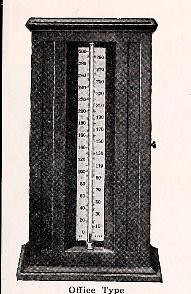This black and white scanned image features a detailed drawing of an old-fashioned office-type thermometer. The thermometer is encased in a tall, wooden box frame. Within the frame, a white placard extends vertically, displaying alternating numerical temperature markings on both sides. On the left, the scale begins at zero and progresses in increments of 20 (0, 20, 40, 60, 80), while on the right, it starts at 10 and moves up by 20 as well (10, 30, 50, 70). 

At the center of the placard, a thin glass tube, presumably containing mercury, rises with temperature changes. The intricate hatching technique used to depict the dark wood of the box frame employs small diagonal lines going in opposite directions, creating a textured, crosshatched appearance. The footnote of the image indicates it is an "office type" thermometer. This illustration appears to be part of a larger scanned document, enriched with fine details and precision.